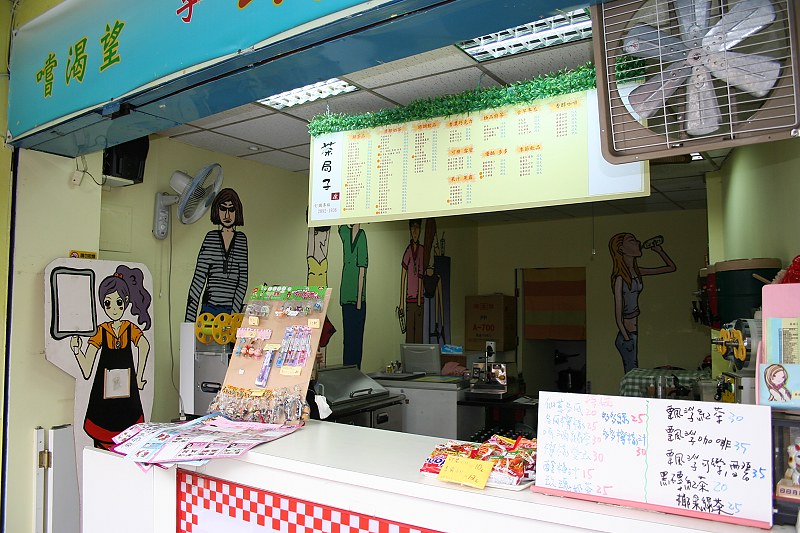The image depicts the front area of a restaurant or cafe, showcasing a vibrant and bustling atmosphere. The foreground features a white checkered counter with red accents, indicating a space where customers can place orders. Behind the counter, a kitchen area is visible, filled with stainless steel cooking equipment and dispensers. Above the counter, a large rectangular menu with Asian characters is prominently displayed, featuring a blue background with yellow and green details and adorned with fake greenery. 

The walls of the establishment are painted yellow and embellished with various colorful cartoon illustrations and drawings of people, including a notable character of a waitress on the left side. Several fans are mounted on the walls, contributing to the restaurant's lively decor. Additionally, other signage and product information written in Asian characters can be seen on a board beside the counter, suggesting an Asian-inspired menu. Furthermore, key rings and other small items are hung on a cardboard stand, adding to the eclectic feel of the place. Overall, the image captures a detailed and vivid snapshot of the restaurant's vibrant front area, highlighting its animated and inviting atmosphere.